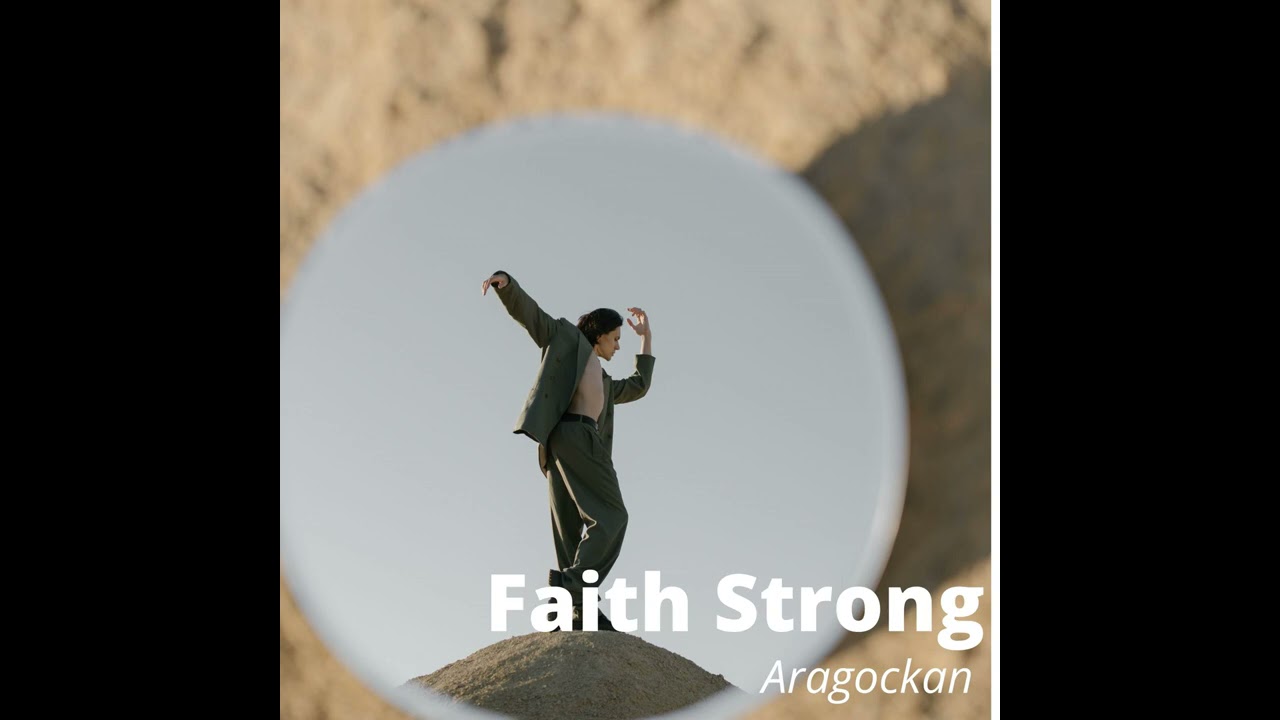The image appears to be the cover of a music album, set against a background of brown sand bordered by black bars on the left and right sides. The focal point is a bluish-gray circle that frames a singular figure standing on a mound of sand or rock. The person, who is likely the musical artist, is of Caucasian descent with shoulder-length brown hair, dressed in a greenish-gray suit paired with a white shirt. They strike a dynamic pose, with the right arm extended backwards and upwards, and the left arm bent in front of them, as if captured in mid-dance. The figure's gaze is directed towards the lower right corner of the album cover, where the name "Faith Strong" is prominently displayed in white text. Below that, in smaller white text, is the possible album title or additional name, "Haro Kakan." The circular frame gives the impression of looking through a microscope or telescope, surrounded by a texture resembling grey concrete or rock.